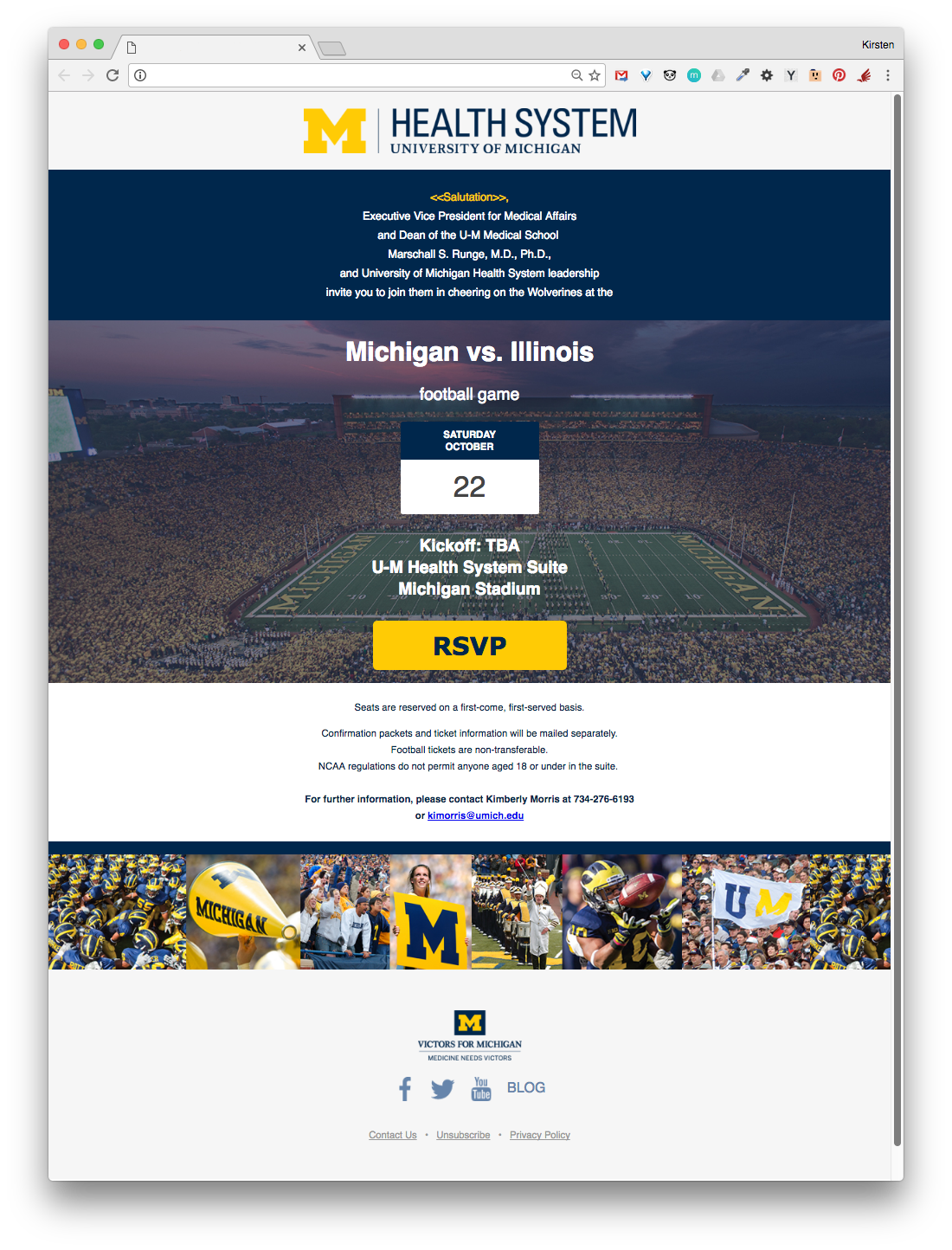At the top of the image, there is a gray rectangle with three circular buttons: a red button on the left, followed by a yellow button, and a green button on the right. Along this gray bar, on the left-hand side, there is an indiscernible symbol, and on the far right, there is an "X" to close the window. Next to the "X," there is a word that is not legible.

Below this bar, there is a navigation section with a left arrow, a right arrow, and a partially visible circular arrow icon. Adjacent to these arrows, there is a search bar—the left side of the bar features a circle with an unknown symbol inside, followed by icons of a magnifying glass and a star on the right. Next to the search bar are various symbols, including:
- The Gmail icon,
- A blue "V" icon,
- A black, indiscernible icon,
- A blue circle with an embedded letter,
- A cloud icon,
- A pen or pencil icon,
- A gear icon,
- The letter "Y",
- An orange and black icon,
- A red outline circle with something red inside, and
- An icon resembling a bird.

Below these symbols, there are three vertically stacked dots, a yellow letter "M," a blue line, and the text "Health System, University of Michigan" in blue. There is a blue rectangle with the top portion in yellow that contains white text, which is too small to read.

Following this, there is an image of a football stadium. At the top of this image, white text reads "Michigan vs. Illinois football game." Below this, there is a blue rectangle with the text "Saturday, October," followed by a white rectangle with "22nd" in black lettering. It also states "kickoff: TBA, U-M Health System suite, Michigan Stadium."

Below this, there is an orange-yellow rectangle with the word "RSVP." Following it is a white rectangle with black text, except for the bottom line, which is in purple. Underneath this section, there is a blue line followed by images related to Michigan football. Further down, there is a blue square containing a yellow letter "M," some blue text underneath, a light blue line, and more text.

At the bottom of the image are icons for Facebook, Twitter, and YouTube, along with the word "blog." Lastly, there are three black words that are not clear.